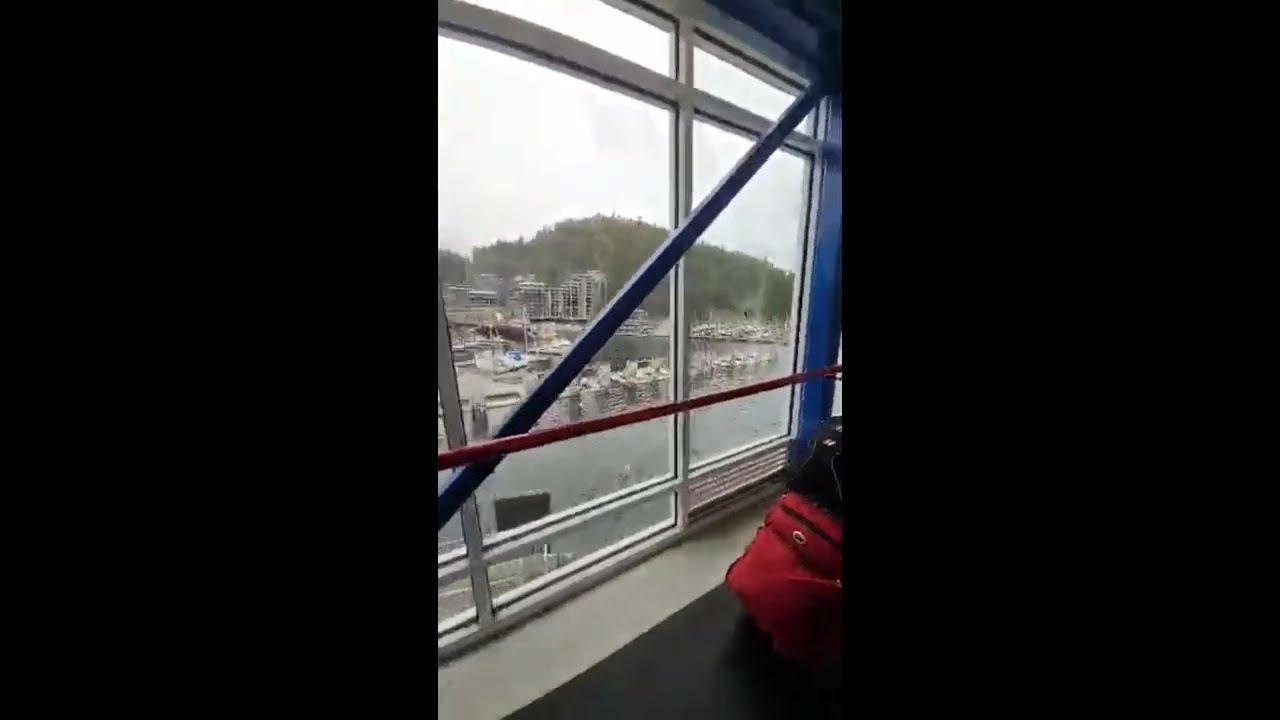The photo, taken vertically with a cell phone, captures a view from inside a building, looking out over a harbor or bay through a window. The window features a distinctive blue diagonal bar and frame, as well as a horizontal red line intersecting the window's white grid. The interior wall where the photo is taken is covered with glass and has a black ledge where a red object, possibly a backpack or elbow of a coat, rests in the lower right corner. The scene outside the window reveals calm, grey water and a distant shoreline with tall white buildings, potentially hotels, and a village-like area nestled against a tree-covered hill. The sky is cloudy, and the overall scene is flanked by black edges on both the left and the right, giving the image a much wider appearance.